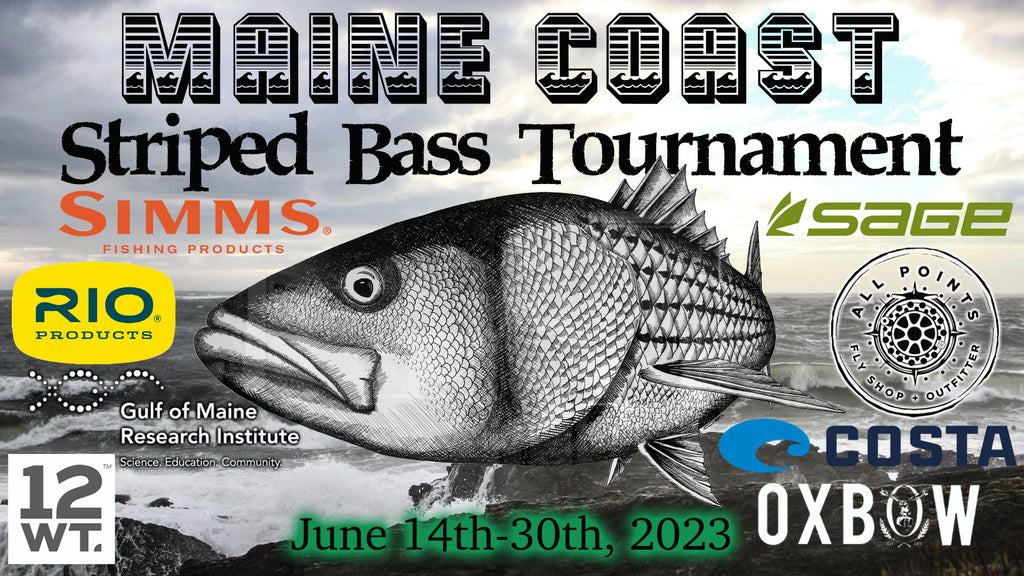This black-and-white advertisement for the Main Coast Striped Bass Tournament prominently features a detailed drawing of a striped bass angled from the right side to the left side. The event, sponsored by numerous organizations including Sims Fishing Products, Rio Products, Gulf of Maine Research Institute, Sage, All Points Fly Shop and Outfitters, Costa Company, Oxbow Company, and possibly the 12WT Company, takes place from June 14th through June 30th, 2023, as stated in bold black letters highlighted in green at the bottom. The backdrop presents an ocean view from the beach, with waves crashing onto rocks under a slightly overcast sky that allows some sunlight to peek through. A variety of sponsor logos in multiple colors—yellow, red, green, and black and white—surround the bass image. Additionally, the bottom left corner features the text "12WT" in a distinct white block.